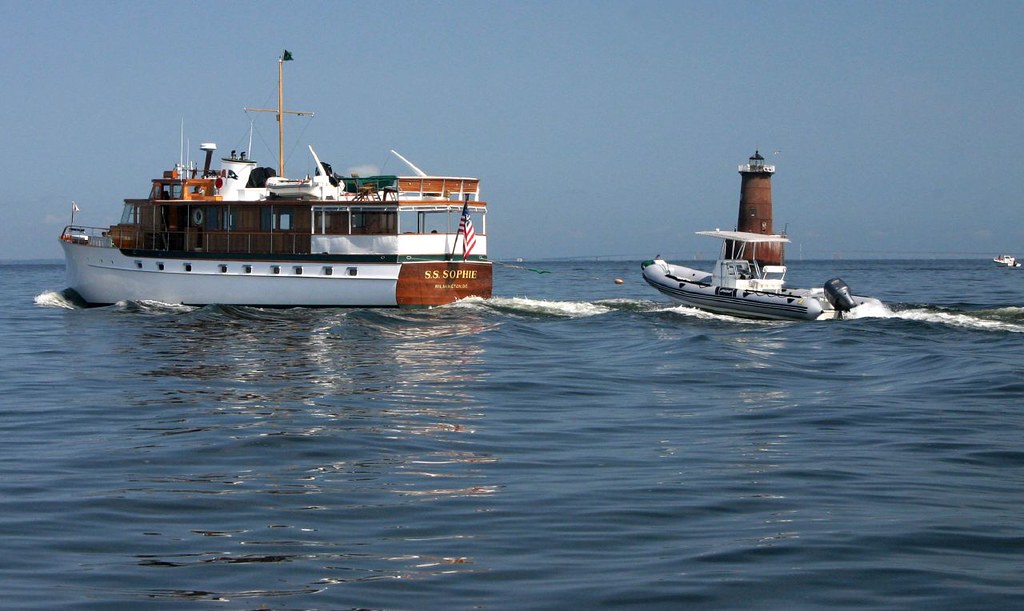This wide rectangular photograph captures a tranquil scene on a body of water, likely an ocean or a large lake. The horizon line is slightly above the center and tilts upwards from left to right under a clear, bluish-gray sky devoid of any clouds. The water, dark blue and faintly rippling, mirrors the boats positioned on either side of the image.

Dominating the middle-left is a larger boat with a white and dark brown wooden body, accented with green portions. This vessel, named "SS Sophie" as indicated by gold lettering over a bright brown wooden section at the rear, also displays an American flag. It heads leftward, slightly tilted, featuring a roof and several sheltered areas. Attached behind it is a small emergency boat.

In the background, to the right of "SS Sophie," trails a smaller white boat, likely a speedboat or fishing craft. Both vessels leave a gentle white wake in their path. Further back, a brick-red lighthouse with a black top punctuates the horizon, contributing a final touch to the serene maritime scene.